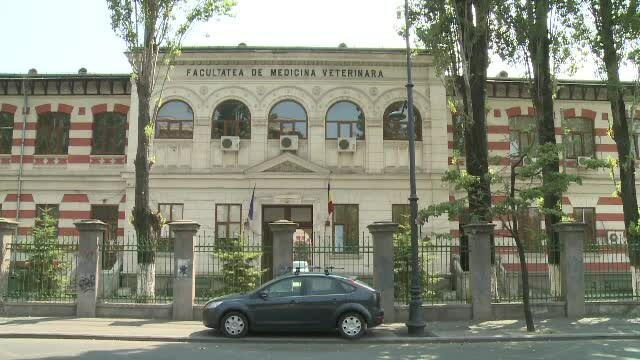The image captures a photograph of an imposing beige stone building, prominently displaying the name "Facultatea de Medicina Veterinaria" across its front facade. The building is framed by wings on either side, which feature striking horizontal red brick stripes. In front of this formal, institutional structure is a high fence composed of cement columns and iron railings, providing a distinct separation from the street. A black hatchback is parked on the sidewalk directly in front of the building. The main structure has three air conditioning units installed in the top floor's central windows, and a triangle pediment crowns the double door entrance. Two flags are mounted on either side of this entrance. The setting is embellished by several large trees, some painted white at the base, and smaller trees, all situated between the fence and the building. The overall atmosphere is one of overcast skies with the sun making a tentative appearance.